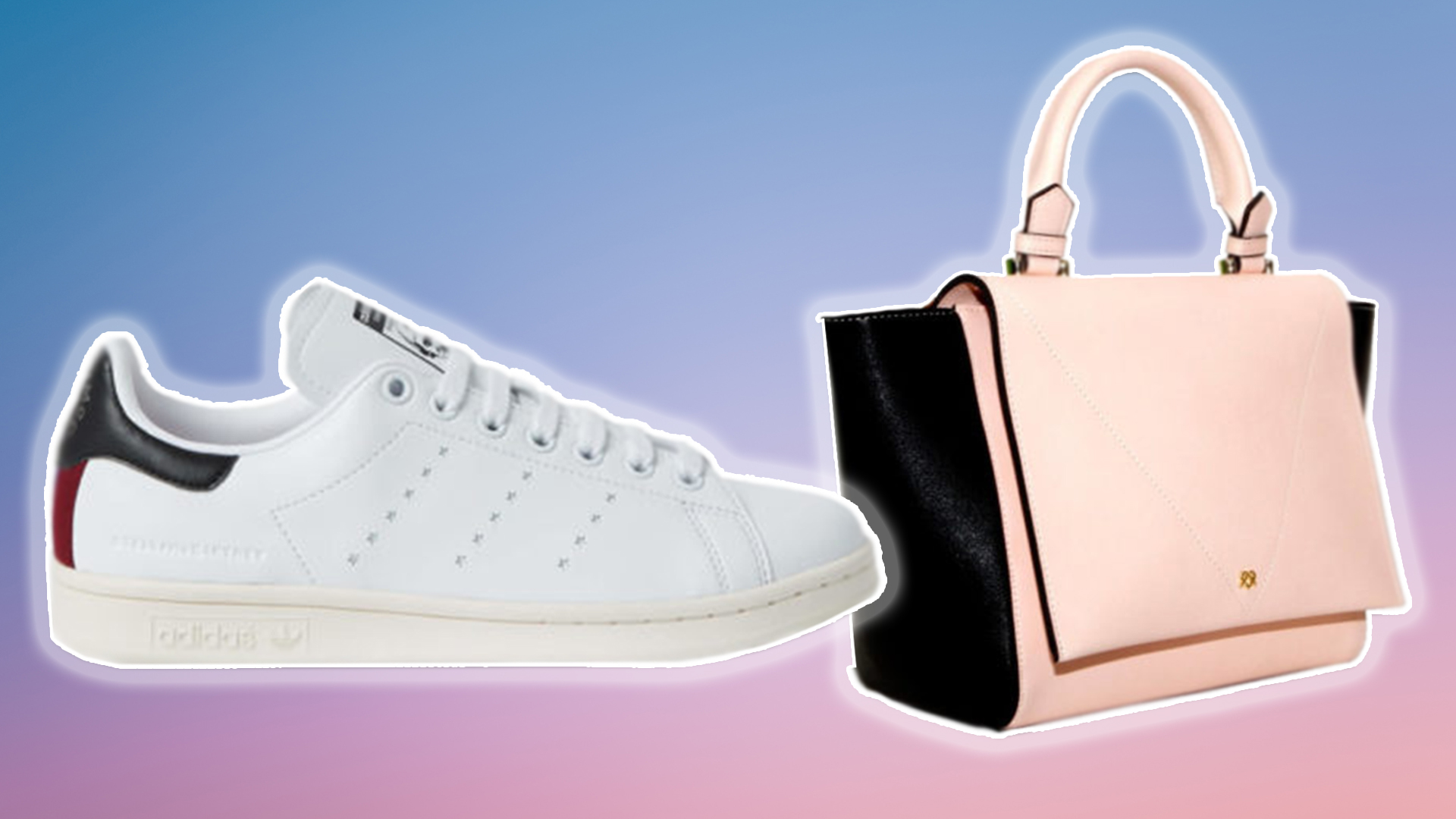The image features a dynamic hologram-like presentation with a striking gradient background, transitioning from a dark blue in the top left to a soft pink in the bottom right. On the left side, there’s an Adidas sneaker, predominantly white with a red vertical stripe and black paneling on the heel, featuring the Adidas logo both on the heel and the sole. The shoe has a white shiny outline with a subtle fading halo effect, giving it a three-dimensional, popping-off-the-screen appearance. To the right, matching in impressive presentation, is a stylish light pink handbag with black side paneling and a short handle. Both the handbag and the sneaker share the same holographic-style white outline and fading halo, enhancing their standout look against the gradient background. The sneaker is oriented with its toe slightly overlapping the handbag, contributing to the overall cohesive and promotional aesthetic of the image.